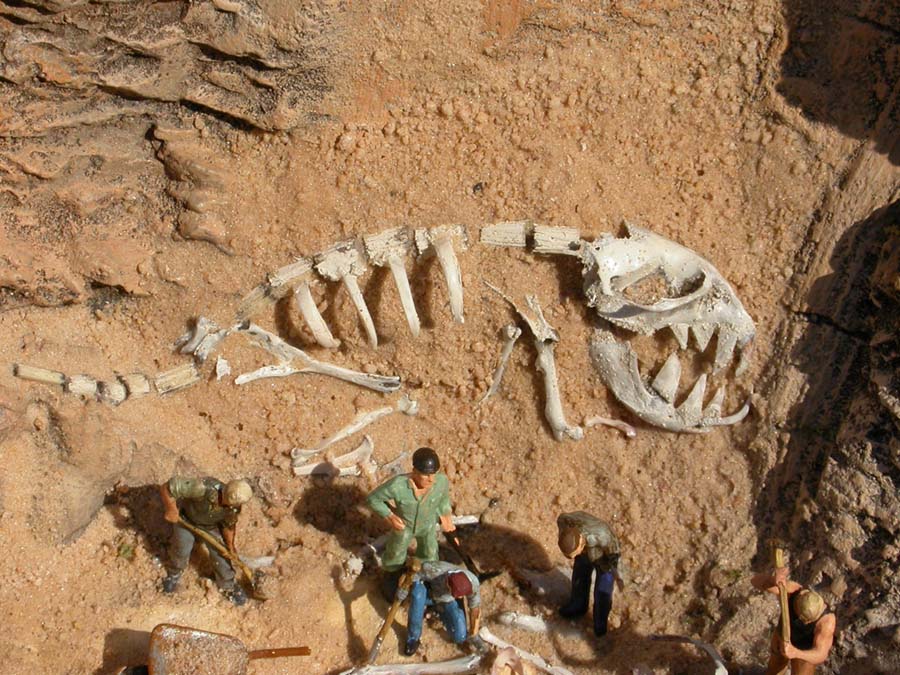This is an overhead shot depicting a dramatic excavation site. Five action figures are meticulously at work in a tan and orange, rocky dirt field. They are uncovering a large, prehistoric dinosaur skeleton. The immense fossil, resembling a creature with a huge jaw and lengthy teeth, stretches across the image from the bottom left, its curved spine and tail extending towards the left side of the frame. The enormous mouth, situated on the right with teeth about a foot long, and hollow eye sockets through which the dirt is visible, dominate the scene. The figures are positioned around the skeleton: one kneeling and one standing upright in a green outfit with a black helmet, another with a shovel on the left, one more mid-dig with another shovel to the right and, at the bottom right, the last figure appears to be working into the rock. The scene is meticulously recreated to illustrate the scale of the uncovered dinosaur bones compared to the action figures, portraying a realistic and detailed archeological dig site.